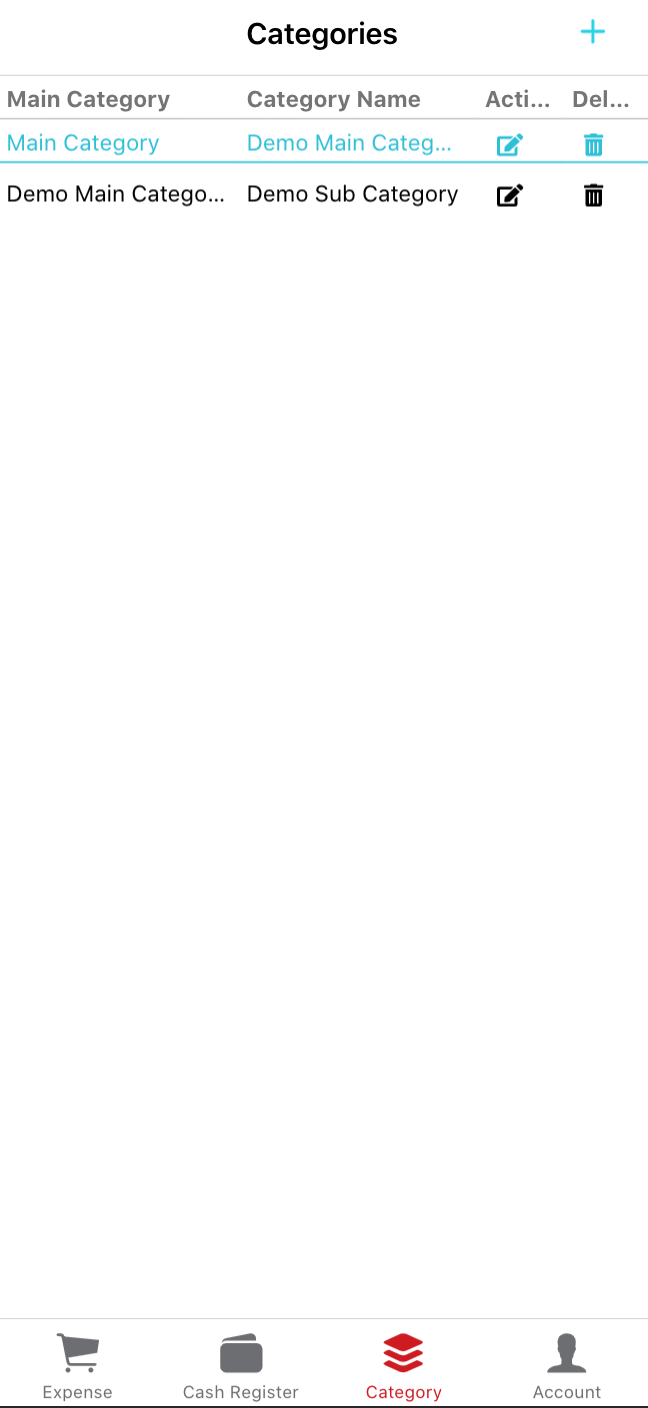Screenshot of a user interface focused on category management. The page is predominantly white, with a "Categories" header. A plus sign icon indicates an option to add a new category. Below the header, there are various columns labeled "Category Name," "Active/Inactive," and "Delete," which likely represent the category details and actions available. The bottom of the screenshot features additional navigation options labeled "Expense," "Cash Register," and "Account," with "Categories" highlighted in red, indicating the currently active section. The design is minimalistic and focused on functionality.